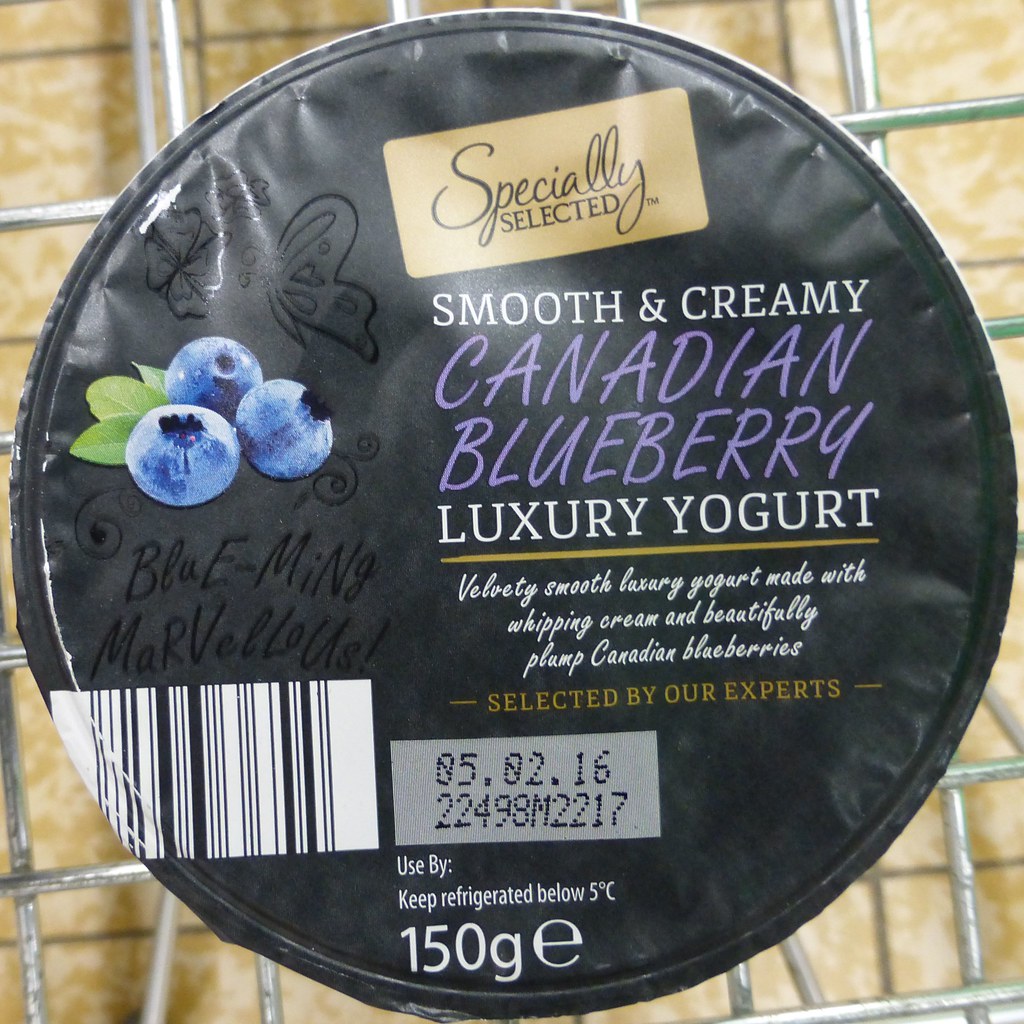This image showcases the top of a black yogurt container. Prominently displayed at the top is a brown rectangle with the text "specially selected." Below this, in purple and white text, it reads "smooth and creamy Canadian Blueberry Luxury Yogurt." The description continues in white script, stating "Velvety smooth luxury yogurt made with whipping cream and beautifully plump Canadian blueberries, selected by our experts." Detailed instructions follow, including a "Best By" date of 05.02.16, a barcode to the left of the expiration date, and storage directions to keep refrigerated below 5 degrees Celsius. Additionally, the container's weight is specified as 150 grams. A realistic depiction of three blueberries with a green leaf is featured on the left side of the container, enhancing its visual appeal. The colors visible in the image include brown, black, purple, blue, green, white, and silver.